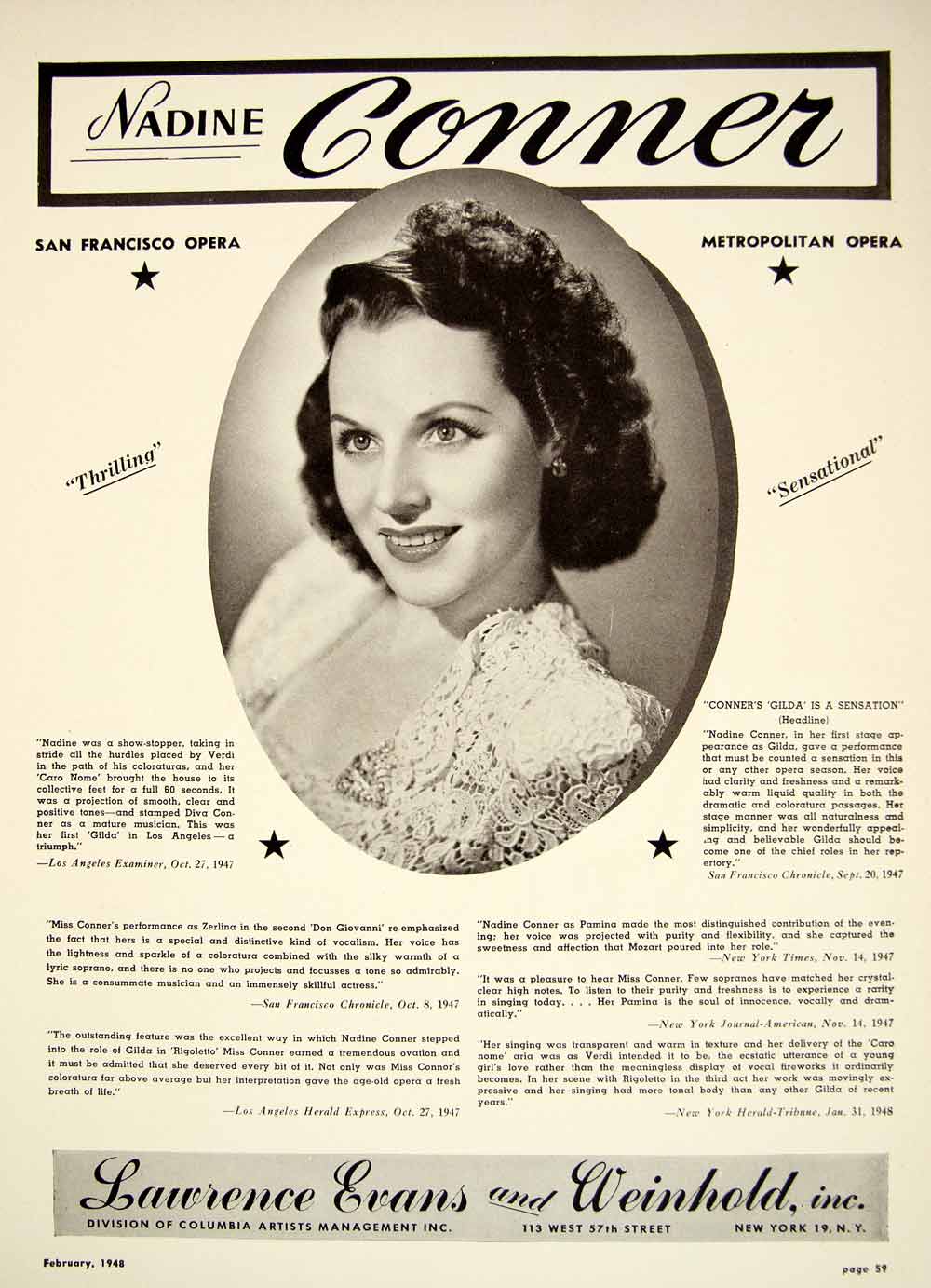This image is a vintage full-page advertisement on aged beige cardstock, likely from a program handout or a 1948 magazine issue. At the top, "Nadine Conner" is prominently displayed in a thick black rectangular frame, with cursive black text. The central portion features a large oval black-and-white sepia-toned photograph of a young woman with wavy, curly hair pulled back from her temples, wearing a lacy dress and looking slightly upward with a smile. Flanking the photograph on either side are phrases promoting her ties to the San Francisco Opera and Metropolitan Opera, along with small text quotations described as thrilling and sensational reviews from notable publications such as the Los Angeles Examiner, San Francisco Chronicle, Los Angeles Herald, New York Herald Times, New York Times, and New York Journal from the 1940s. The bottom half of the page contains two columns of text and pull quotes surrounding the image. A gray banner at the very bottom spans the width of the advertisement, with cursive text reading "Lawrence Evans and Weinhold Inc." and smaller text beneath that noting "Division of Columbia Artists Management Inc., 113 West 57th Street, New York, 19 New York." Additionally, the date "February 1948" and "page 59" are marked in small print on the left and right corners of the bottom section, respectively.